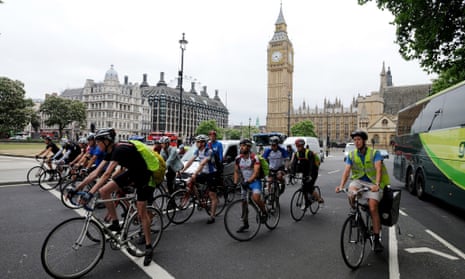The image depicts a bicycle race during daytime, characterized by an overcast sky. The cyclists, closely packed and ready to race, are poised at the starting line, mounted on bicycles with black tires and wearing varied jerseys in colors such as black, green, blue, and red. Each cyclist is equipped with helmets and additional biking gear, including shoes, and some are seen sporting bright yellow vests over their outfits.

From a slightly side-on perspective, the racers are situated on a dark gray pavement. They appear prominently at the lower half of the image, particularly towards the left and middle sections. Just to the right of the scene is a parked bus with a black and green body.

In the background, historic landmarks, including tall old buildings of gray and light gray concrete, dominate the skyline. A distinctive golden clock tower reminiscent of Big Ben is notable. To the left is a white building, while trees and foliage can be seen extending into the top right corner of the frame. This scene captures the blend of competitive sports against a backdrop of urban architecture and historic monuments.